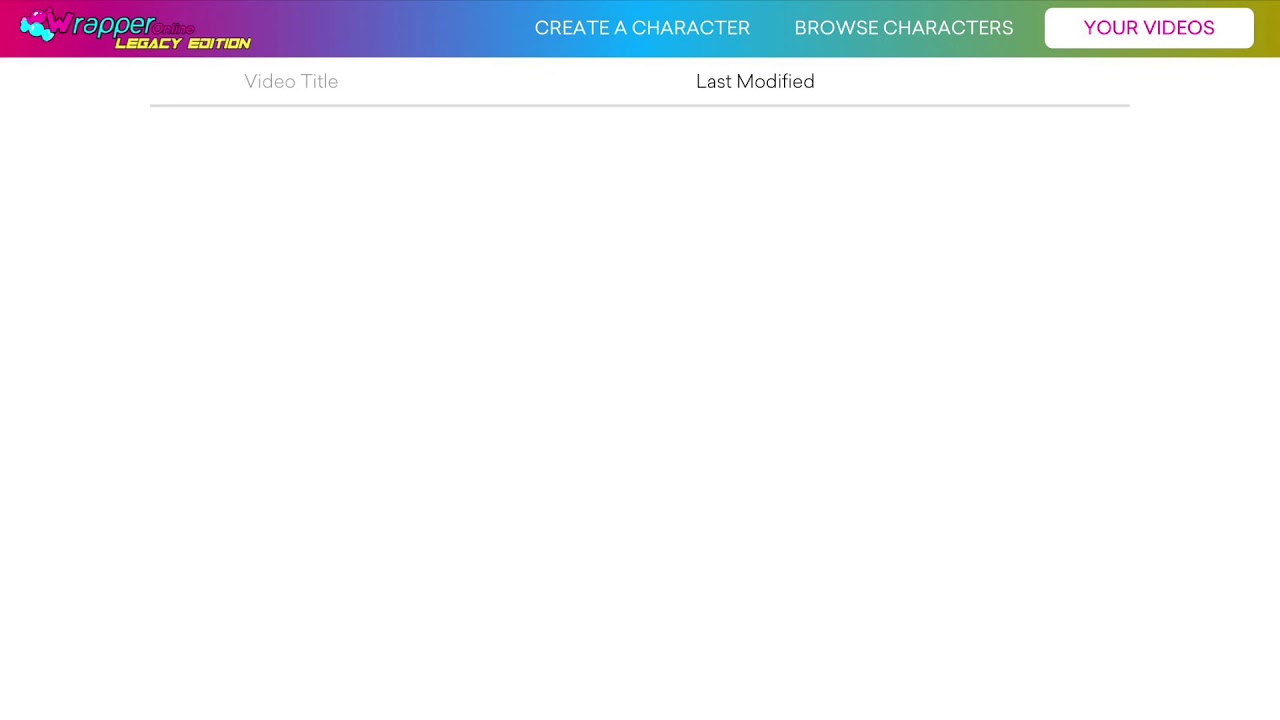The image depicts a webpage header bar, presumably from a website named "Wrapper Online: Legacy Edition." The design is vibrant, showcasing a pink 'W' in 'Wrapper' followed by 'rapper,' spelled out in blue. The background of the header features a dynamic color gradient transitioning from pink-purple on the left, through blue, and into green, with a slight hint of yellow-green at the far right.

The header includes navigational options such as "Create a Character," "Browse Characters," and "Your Videos." Below these options, there are sections labeled "Video Title" and "Last Modified," which currently show no entries, suggesting that the user logged into their account has not uploaded any videos yet. Despite the lack of uploads, the presence of a "Your Videos" section confirms that the person has created an account on this website.

The logo of "Wrapper Online" is accentuated by two candy wrapper icons, one in pink and the other in blue, though it does not provide much additional context about the site's purpose. The overall interface indicates a web platform where users can likely create and share character-based video content.